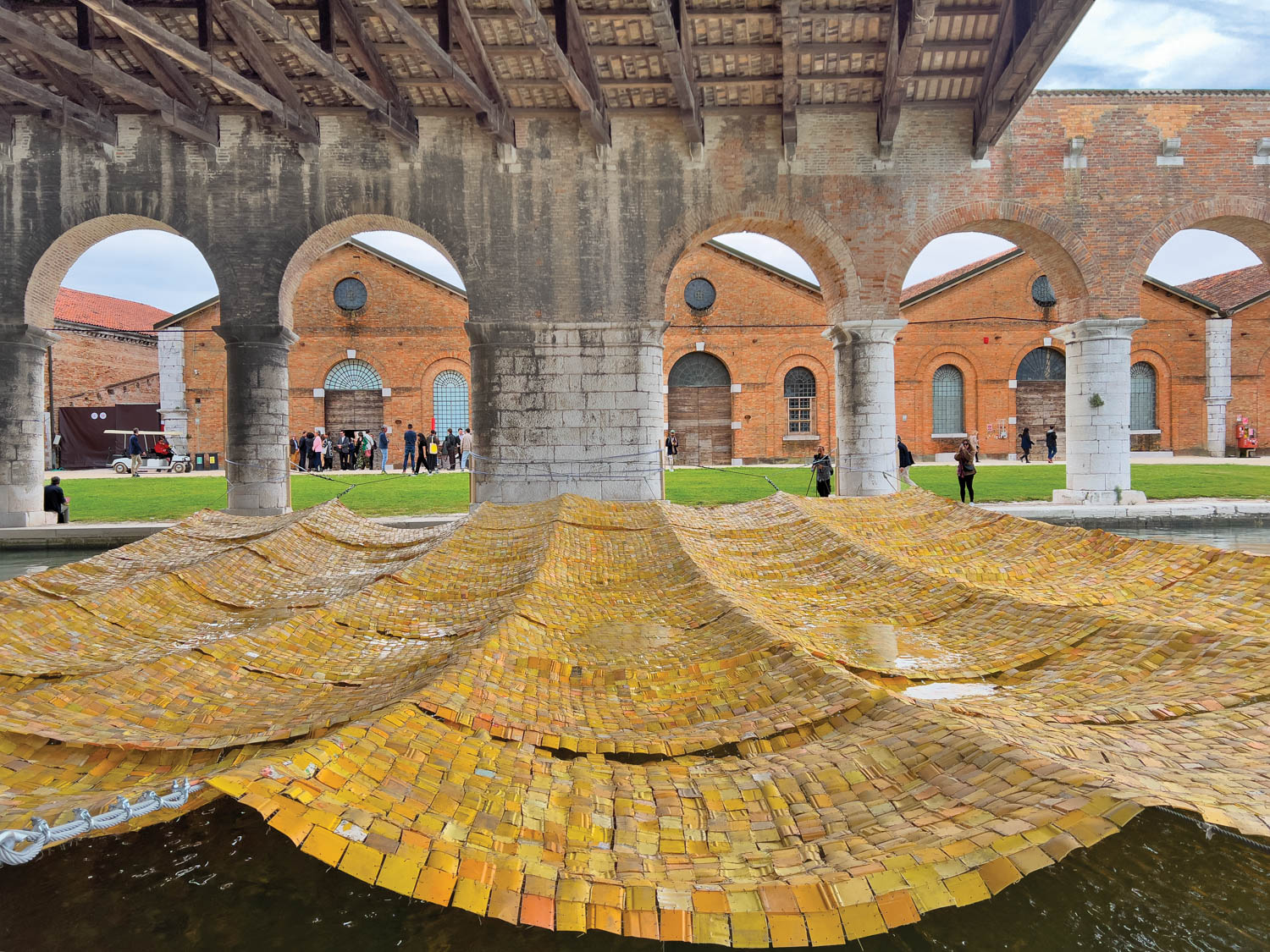In this outdoor photograph, the central focus is a large, intricate tapestry made up of thousands of small squares, predominantly yellow, interspersed with whites, browns, and reds. The tapestry, which resembles a corncob due to its repeated square patterns, is suspended by ropes over a waterway and stretches from the bottom to the midsection of the image. This artistic installation is held up by pillars, and through the open arches of these pillars, we glimpse a green grass lawn leading to a sidewalk and several brick buildings in the distance. These buildings feature arches, wooden doors, and windows, and a white golf cart is parked nearby. Many people are gathered around the tapestry and the buildings, some taking photos of the vibrant scene. The arches and the open-air structure suggest a courtyard setting, possibly at a school or public area, creating a picturesque and communal atmosphere.